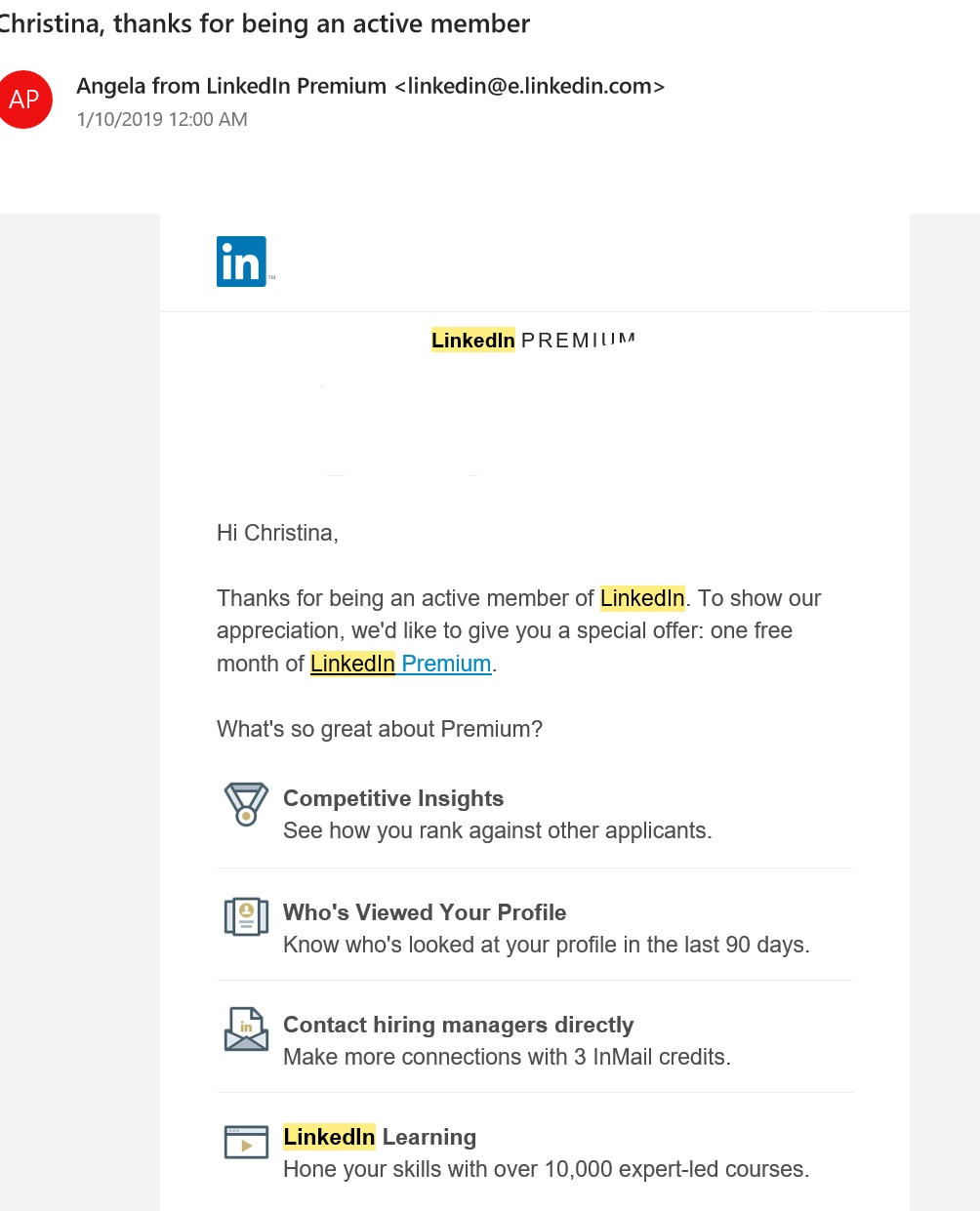This is a screen grab of a LinkedIn webpage. At the top, there is a personalized greeting that says "Christina, thanks for being an active member." Below this, there is a red circle with a white "AP" inside it, and adjacent to the circle, there is text in black that reads "Angela from LinkedIn Premier" with a small "LinkedIn" logo followed by the email address "e.linkedin.com." The timestamp provided is January 10, 2019, at 12 a.m.

The main body of the webpage appears as though it resembles a letter or a promotional message. It opens with "Hi Christina," followed by a thank you message for being an active LinkedIn member. The message goes on to offer Christina a special deal: one free month of LinkedIn Premium. The perks of LinkedIn Premium highlighted in the message include:

- **Competitive Insights:** See how you rank against other applicants.
- **Who's Viewed Your Profile:** Know who has looked at your profile in the last 90 days.
- **Contact Hiring Managers Directly:** Enhance your networking with three InMail credits.
- **LinkedIn Learning:** Access to over 10,000 expert-led courses to hone your skills.

The references to "LinkedIn" throughout the page are highlighted. The overall layout of the page shows a thicker gray border on the left side compared to the right, which is also gray. In the top left-hand corner, there is a blue square with a white "IN" logo, indicating the LinkedIn branding, and appears clickable. The webpage is not perfectly centered, adding to its distinct design elements.